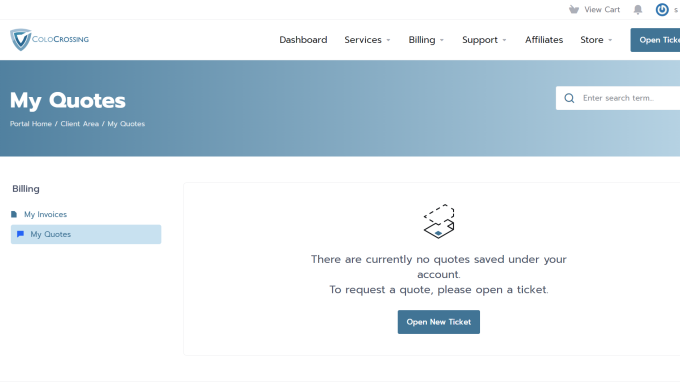This screenshot from the Cold Crossing website displays various elements that make up its user interface. At the top left corner, the website's title is prominently positioned. Adjacent to it, a menu bar includes options such as Dashboard, Services, Billing, Support, Affiliates, and Store. Above this menu bar, a blue "Open Ticket" button is available. The status bar features a view cart icon and a notification bell icon.

Immediately below the main navigation, a section titled "My Quotes" is set against a blue background. On the far right of this section, there is a search bar for user convenience. Moving down, the primary content area of the webpage is mostly white, with a sidebar on the left. The sidebar contains categories such as Billing, and within Billing, subcategories like My Invoices and My Quotes. The "My Quotes" section is highlighted in blue.

The main content area, on the right side of the page, displays a message box taking up a substantial portion of the space. This box informs the user that there are currently no quotes saved under their account. To request a quote, users are prompted to "Open a Ticket," with another blue "Open New Ticket" button provided below the instructional text. Above this message, there is an icon depicting a piece of paper layered over another outlined piece of paper, symbolizing documents or quotes.